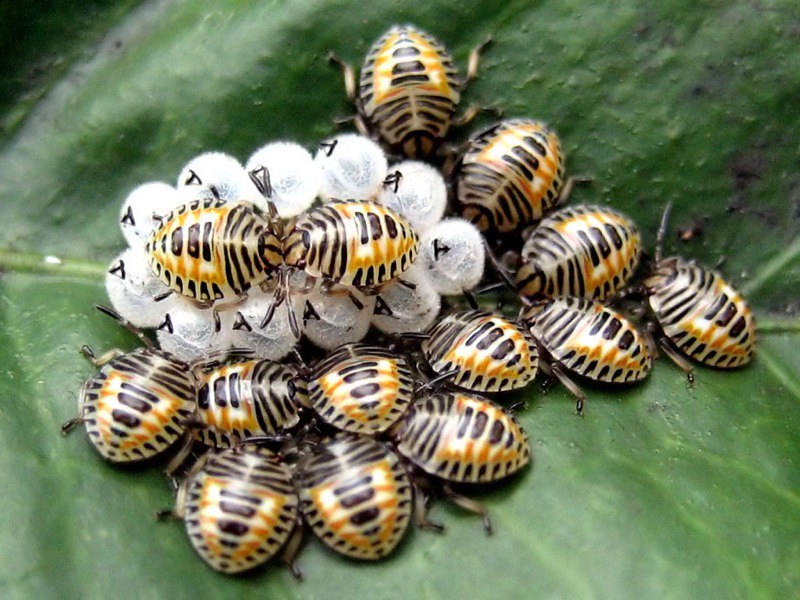This vibrant color photograph captures a close-up view of approximately a dozen small beetles, each about the size of a ladybug, congregating on the center of a dark green, glossy leaf. The leaf is oriented with the bottom to the left and the top pointing right, though neither end is visible in the frame. The beetles, identified by their hard shells, exhibit a unique striped pattern with colors ranging from cream and black to orange and yellow. They have cream-colored heads and thoraxes with black stripes, while their abdomens feature interrupted black lines over an orange background with cream highlights. Their black legs and antennas are also prominent. These beetles are clustered around what appears to be a clutch of around 11 translucent, white eggs with slight transparency, some with tiny black spots. The leaf’s prominent center vein and radiating smaller veins accentuate the setting. This image, taken with a regular camera, creates a detailed and dynamic scene of beetles seemingly jostling for space around their eggs on the shiny green leaf.